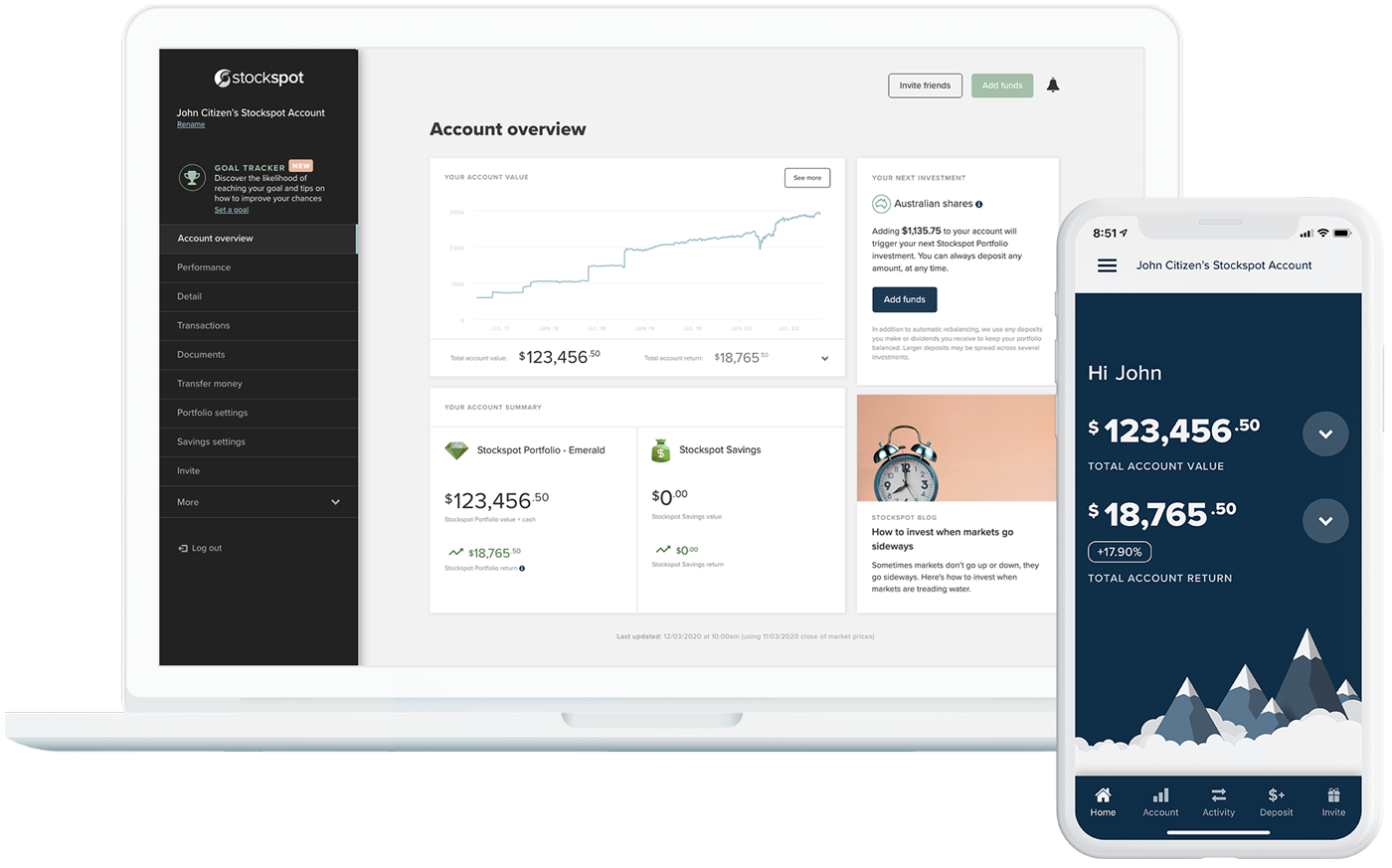This detailed caption describes two related images showcasing the account information of an individual named John Crone. 

The first image appears to be a screenshot from a tablet displaying a webpage for an investment platform called "Stock Spot." The page features an "Account Overview," indicating that it provides users with the ability to purchase, sell, and manage stocks. The account in focus belongs to John Crone and shows a total balance of $123,456. This overview seems to include detailed information about the account's stock holdings and investments.

The second image, positioned to the right of the tablet screenshot, is a capture from an iPhone displaying a related app interface. The app also belongs to John Crone, as indicated by the greeting "Hi John" and mirrors the same total account value of $123,456. Additionally, it provides an overview of the account's total return, which amounts to $18,765. This suggests that the iPhone app offers an easy way to view detailed financial summaries and track investment performance.

Together, these images demonstrate how John Crone manages and monitors his investments through both a tablet and an iPhone application for the "Stock Spot" platform, highlighting the synchronization and accessibility of his financial data across multiple devices.